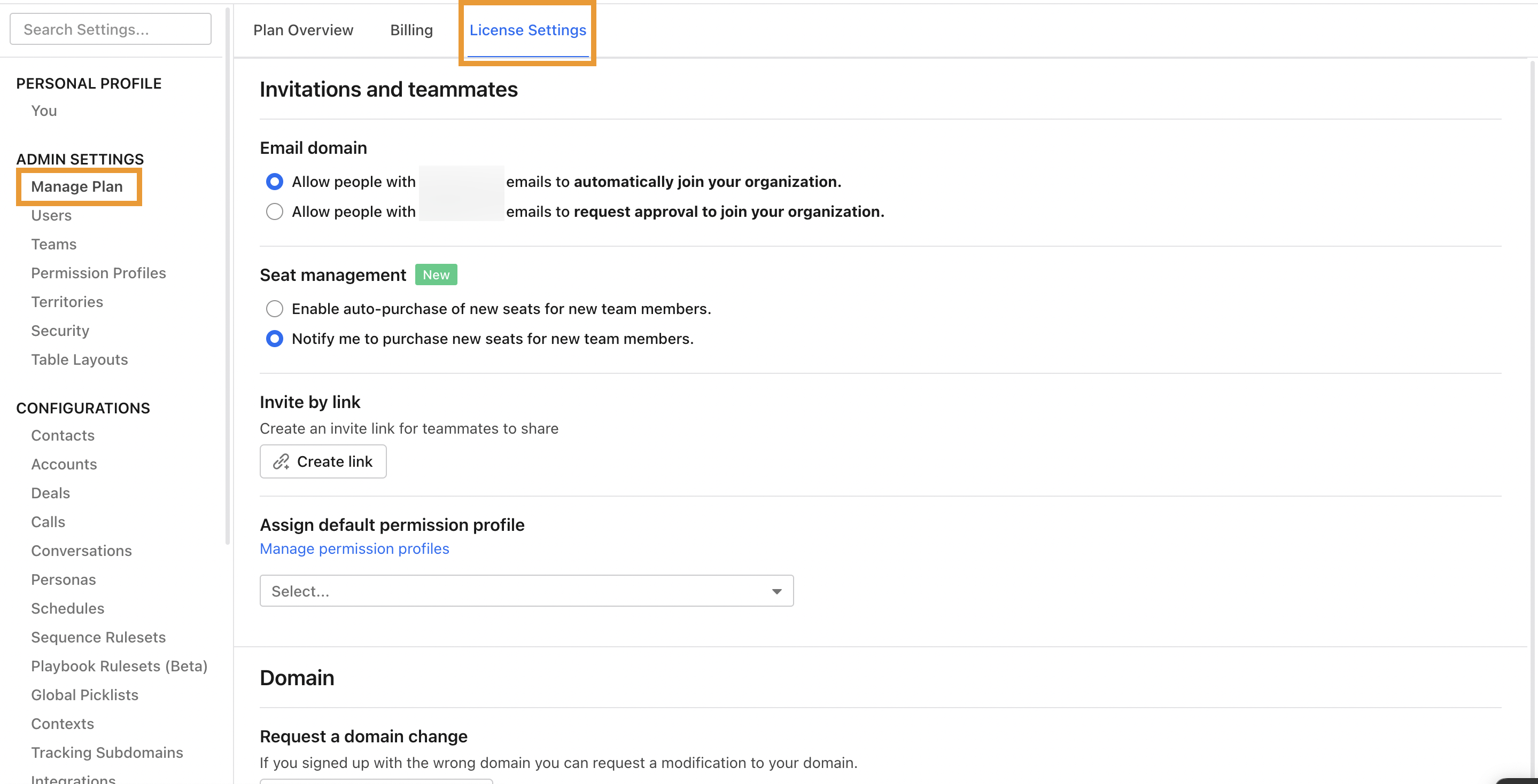The website menu is presented as a vertical column on the left side of the screen. At the top of the column, there is a section for "Search Settings," followed by the "Personal Profile" header, which includes user details. Below this, another header labeled "Admin Settings" is displayed. Under "Admin Settings," various options are listed:

- "Manage Plan" (highlighted with an orange box indicating it is currently selected)
- "Users"
- "Teams"
- "Permission Profiles"
- "Territory"
- "Security"
- "Table Layouts"

Further down is a "Configurations" section with the following options:

- "Contacts"
- "Accounts"
- "Deals"
- "Calls"
- "Conversations"
- "Personas"
- "Schedules"
- "Sequence Rule Sets"
- "Playbook Rule Sets"
- "Beta"
- "Global Pick List"
- "Contacts"
- "Tracking Subdomains"
- "Integrations"

The main content area on the right side of the screen shows detailed settings and options for the "Manage Plan" section, which include:

- "Plan Overview"
- "Billing and License Settings" with "License Settings" selected
- "Invitations and Teammates"
- "Email Domain" with a note about allowing people with certain email addresses to automatically join the organization
- "Seat Management"
- "Invite by Link"
- "Assign Default Permission Profile"
- "Domain"

This detailed structure offers an organized view of the website's menu and its various functionalities, clearly demarcating administrative and configuration settings from user profile options.